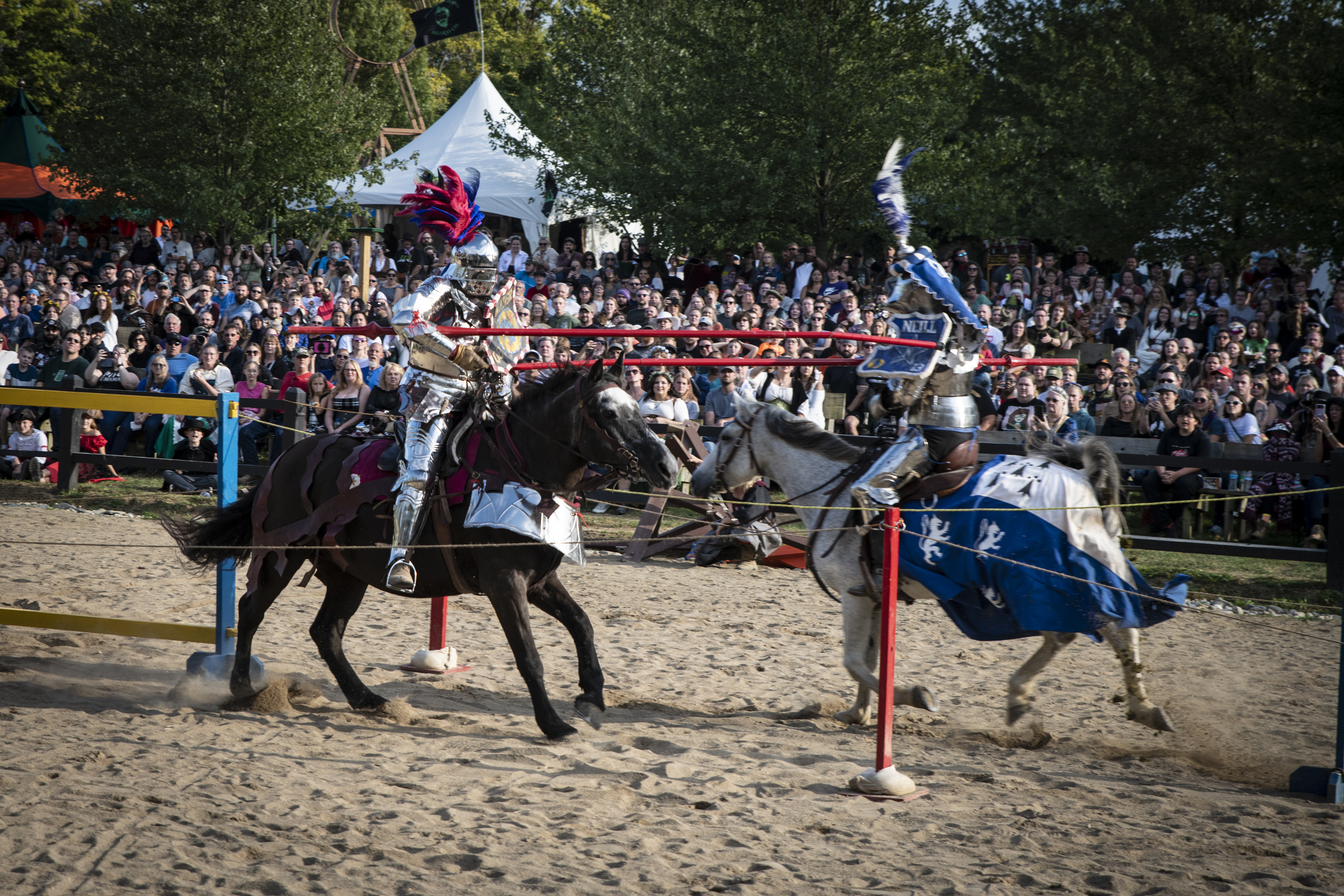This image depicts a lively jousting tournament, likely set at a renaissance fair or festival. Two knights, fully adorned in shiny silver armor, are mounted on horseback, poised to duel. The knight on the left rides a dark brown horse, and adorns red and blue feathers on his helmet while holding red jousting poles. His opponent on the right rides a white horse, which features a blue and white covering. This knight has white hair and is adorned with a white feather on his helmet. Both knights are positioned in a sandy arena, with a small fence separating their paths. A large crowd of spectators fills the stands in the background, adding bustling energy to the scene. Behind the spectators, a lush green expanse of trees and a white triangular-roofed tent can be seen, completing the festive atmosphere.